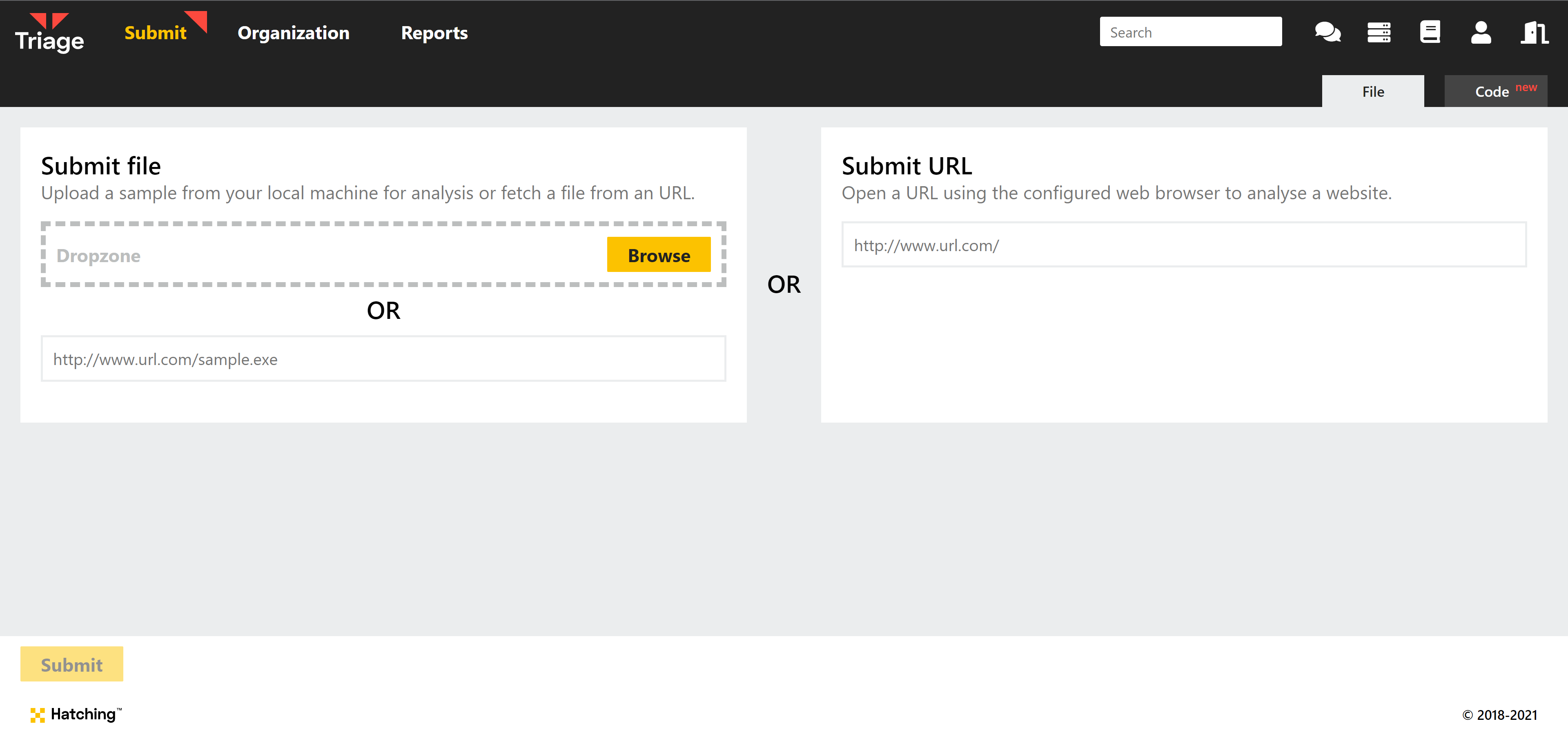The image depicts a website interface with a black navigation strip across the top. In the upper left corner of this strip, the word "Triage" is displayed in white text, accompanied by two red triangles above it. On the right corner, the word "Submit" appears in yellow, with a single red triangle above it. The words "Organization Reports" are shown in white. To the right side of the navigation strip, there is a white search bar.

Below the navigation strip, various icons are displayed, including white text bubbles, a disk icon probably representing a save function, a person icon, and another unidentified icon. There are two tabs labeled "File" and "Code New." The "Code New" tab is gray with the word "NEW" in red and "CODE" in white. The active tab is "File."

Under the "File" tab, instructions are provided to "Submit File." Users are prompted to either upload a sample from their local machine for analysis or fetch a file from a URL. There's a "Drop Zone" area and a yellow "Browse" button with black font for selecting a file. Users can also input a website address in a data bar, which displays an example format.

The section also provides an alternative option, marked by the word "OR," which offers to "Submit URL." This allows users to open a URL using the configuration web browser to analyze a website. An example URL (http://www.url.com/) is shown in the data input field.